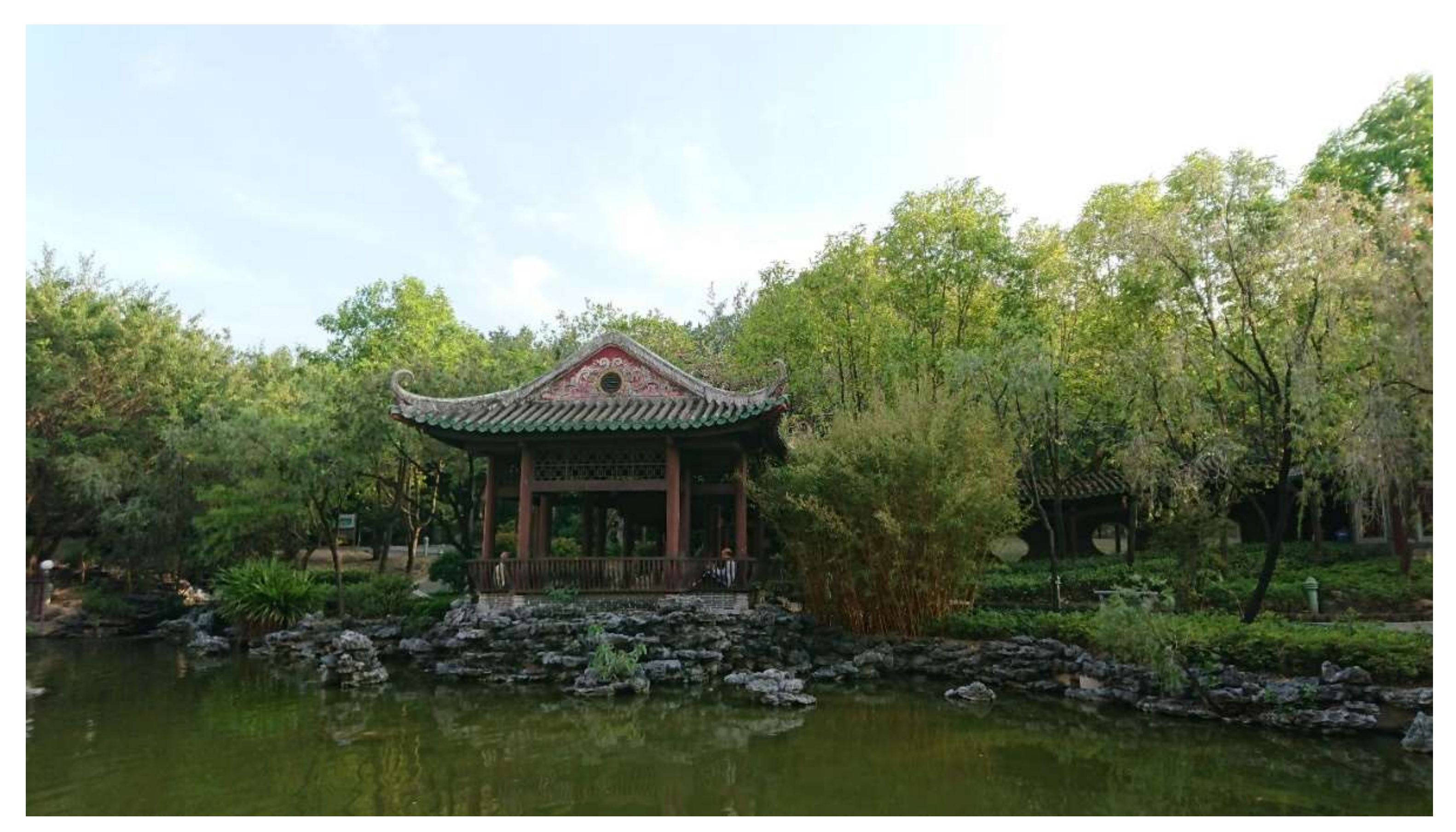The image presents a detailed and vibrant scene, likely modeled on an Asian architectural and natural aesthetic. It features a picturesque landscape dominated by a white sky that serves as a serene backdrop to the lush greenery below. Spanning the width of the image are green trees with brown stems and branches, interspersed with red and brown hues, particularly on the left side near a housing area, and lighter green tones on the right.

In the back right, a brown housing structure can be spotted, while more centrally situated, slightly to the left, stands a red building resembling a gazebo with a distinctive green roof and brown railing. This structure has an air of traditional Asian design, possibly serving as a communal or meditative space within a garden setting. This gazebo appears to signal some cultural significance, accentuated by what seems to be a small statue or bust within it.

The foreground is marked by a tranquil pond, its water a murky green, bordered by an array of rocks in varying shades of gray, black, and tan. On either side of the pond, people are visible, one dressed in yellow and the other in blue, seemingly enjoying the peaceful environment. The scene is enriched with gardens brimming with diverse plants and rock formations, contributing to the overall ambiance of tranquility and cultural reverence.